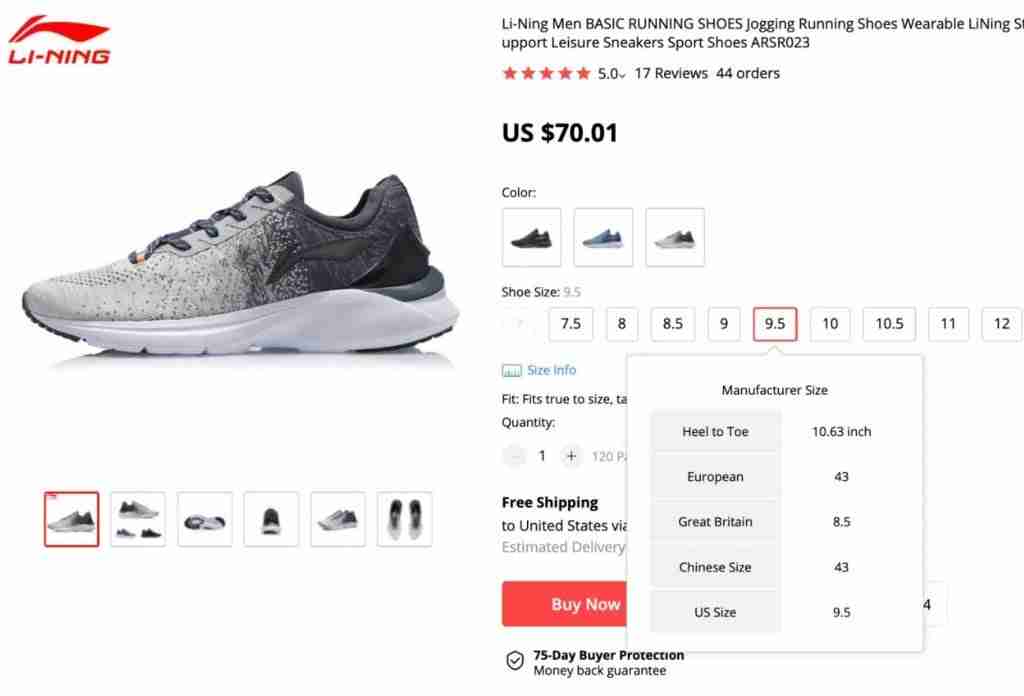The product page features Li Ning (L-I-N-I-N-G) Men’s Basic Running Shoes, model ARS R023. The running shoe boasts a stylish design with a white sole and a gradient upper that transitions from light gray at the front to a charcoal blue and gray toward the back. Prominently displayed in the upper left-hand corner is the red logo of the Li Ning brand.

Touted for its comfort and versatility, the shoe is described as "Leaning Men's Basic Running Shoes, Jogging Running Shoes, Wearable Leaning Support Leisure Sneakers Sport Shoes." The product enjoys a high rating of 5 stars based on 17 reviews and has been ordered 44 times. Priced at U.S. $70.01, the shoe size currently displayed is 9.5, along with conversion details for various international sizing standards, including European, Great Britain, and Chinese sizes. Detailed equivalent measurements from heel to toe are also provided to assist in selecting the correct fit.